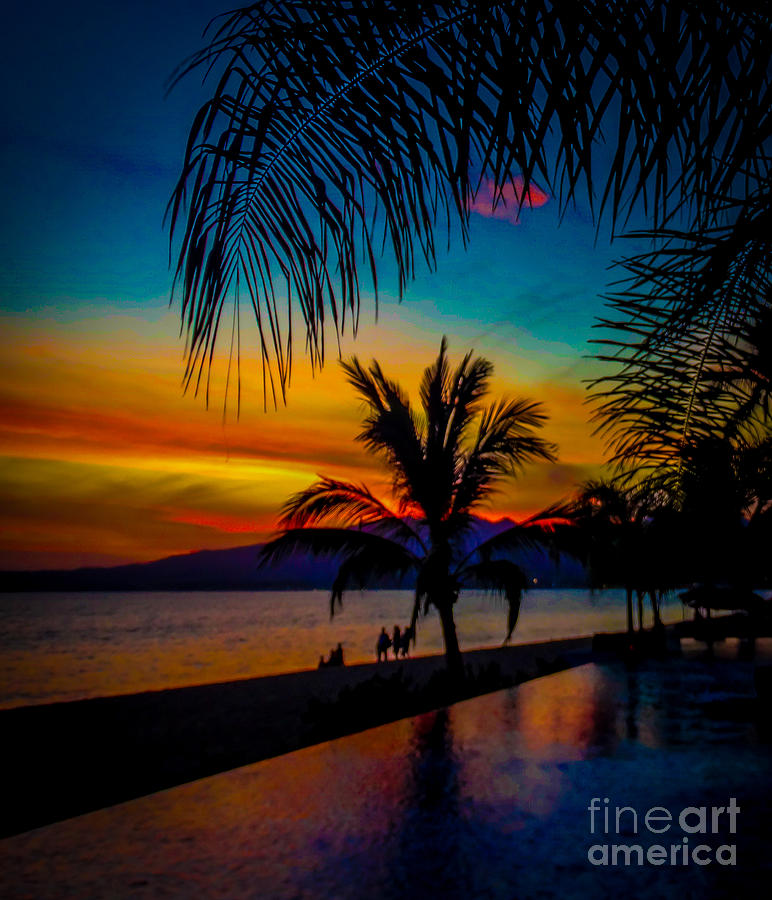This photograph captures a serene tropical beach at sunset, featuring a stunning gradient sky. The top of the sky is a deep turquoise blue, transitioning through lighter blue and pinkish-orange to vivid orange and yellow hues near the horizon, highlighting the setting sun. A majestic mountain range dominates the background, hinting at a location like Hawaii. Below the mountains, the ocean reflects the brilliant colors of the sky. In the foreground, a small beach area hosts four individuals, their shadows cast long on the sand. The centerpiece of the image is a palm tree standing tall, with another palm tree's leaves framing the top right corner. A shiny, potentially reflective surface, possibly a piece of tile or concrete, appears in the bottom right corner. The photograph is marked with "Fine Art America" in the bottom left, underscoring its artistic value.